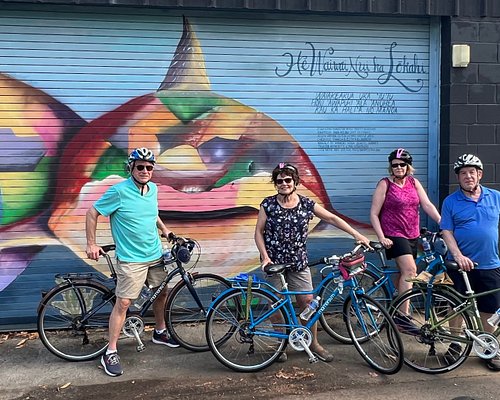This image captures a vibrant scene of four middle-aged Caucasian bicyclists posing in front of a large, commercial garage door adorned with a colorful mural. The mural depicts a multi-colored sea creature, possibly a whale or shark, with a blue background. The creature stands out in vivid hues of red, green, orange, yellow, pink, and beige, featuring a distinct mouth, two eyes, and what appears to be a fin or horn at the top. There is some non-English writing in blue cursive at the top right, along with smaller text beneath it. 

The four individuals, all equipped with helmets and sunglasses, exude positivity with their cheerful expressions. On the far left, a man in a teal shirt, khaki shorts, and gray sneakers with white laces stands over his black bike. Beside him, a woman with short hair is dressed in a black patterned blouse and khaki shorts, holding onto her blue bike. Slightly behind her, another woman sports a hot pink patterned shirt and a black helmet with a pink stripe, standing beside her blue bike. The man to her right wears a blue collared shirt and a whitish-black helmet, standing behind his green bike with its saddle held in his hand. Scattered leaves add a touch of nature to the sidewalk where the group stands.